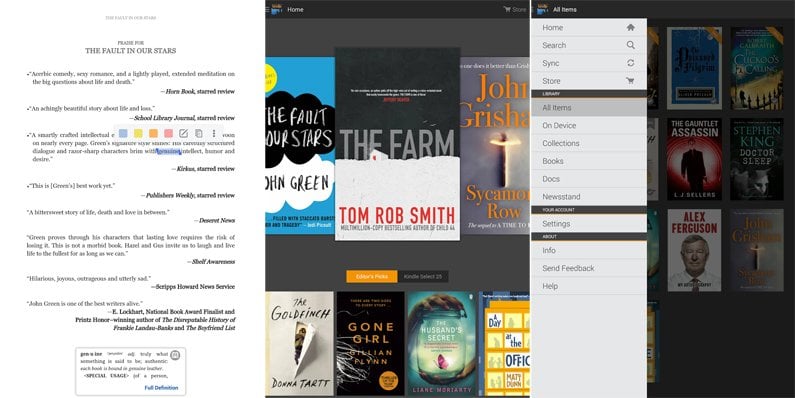The image features a comprehensive display divided into two main sections. 

On the left side, there is a highlighted segment titled "Praise for The Fault in Our Stars," showcasing various quotes from different reviewers. This section uses color highlights to draw attention to specific parts of the text. Additionally, there is a bar at the bottom of this section with various colors, alongside a small box that prompts for a full description.

The right side of the image displays a collection of book covers and titles. Prominently featured is "The Fault in Our Stars." Other books displayed include "The Farm" by Tom Robb Smith, "Sycamore Row" by John Grisham, "The Goldfinch" by Donna Tartt, "Gone Girl," "The Husband's Secret," and "A Day at the Office." 

In addition, there is a multi-screen layout on the right. The last screen reveals a gray navigation bar at the top with options labeled "Home," "Search," "Sync," and "Store." Under the "Library" category, it displays options such as "All Items," "On Device," "Collections," "Books," "Docs," and "Newsstand." Further options include "Your Account," "Settings," "About," alongside information sections labeled "Info," "Send Feedback," and "Help."